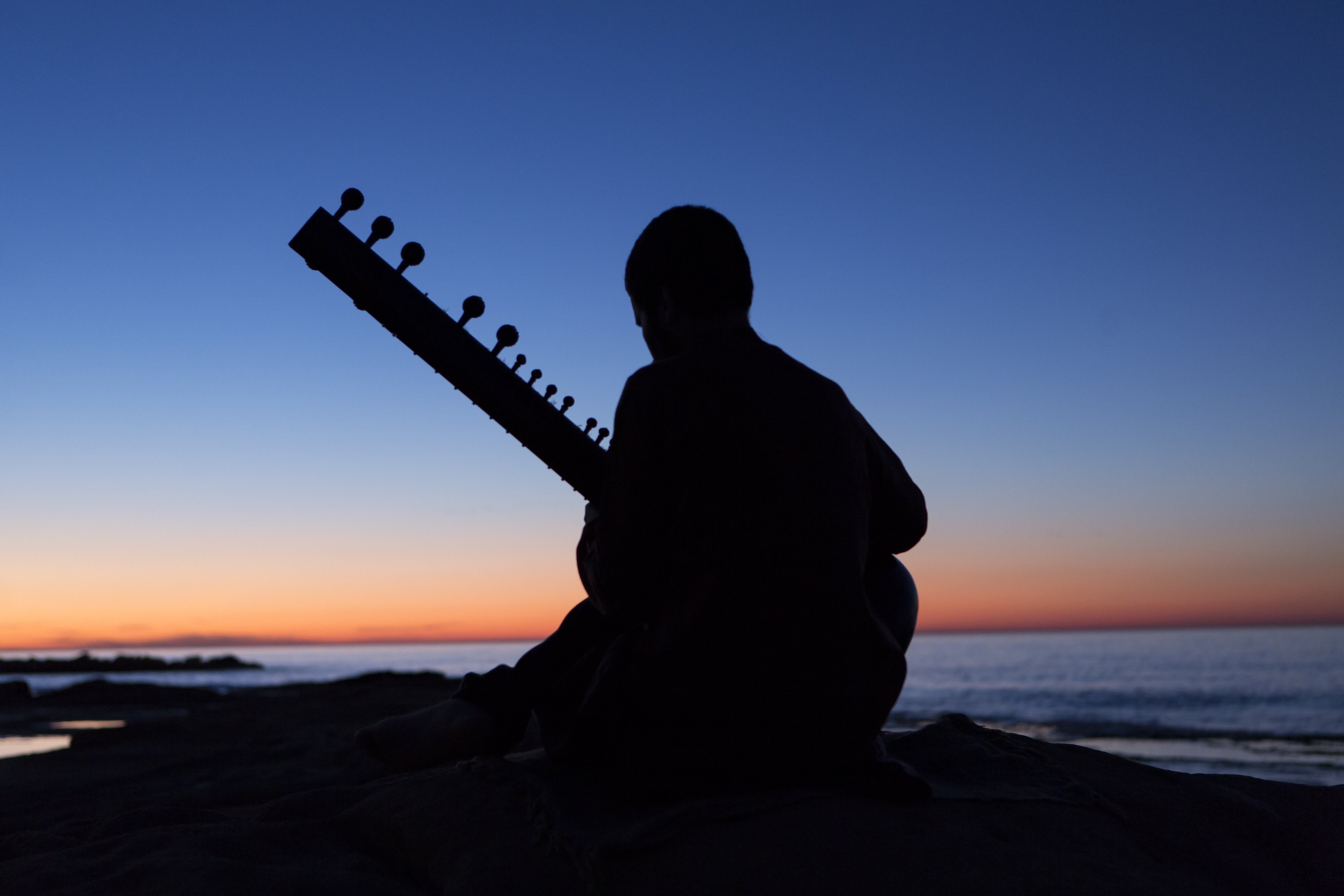In this rectangular color photograph taken at dusk, a person sits on a rocky outcrop by the calm, bright blue water. The serene scene captures the golden moment just past sunset, where the horizon glows with vivid streaks of pink, orange, and yellow, gradually transitioning into a deep, cloudless blue sky. The individual sits with their back to the viewer, silhouetted entirely in shadow, making detailed features, such as gender or ethnicity, indiscernible. The person appears to have short hair and is engrossed in playing a large, stringed instrument resembling a sitar or an elongated guitar, characterized by its long bar and multiple tuning knobs. The tranquil water at the base of the rocks reflects the last light of the day without any disturbance, creating a harmonious and peaceful atmosphere.